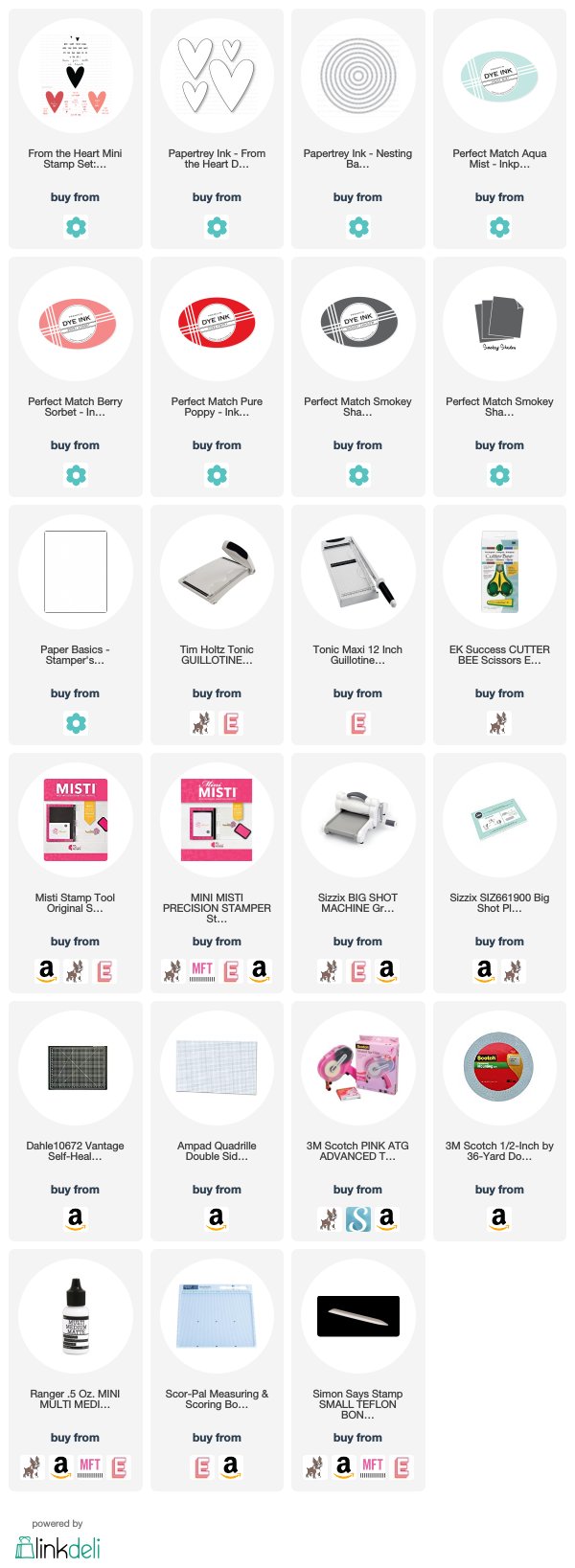This image from an unknown website showcases a variety of crafting and stamping supplies organized from top to bottom. Here's a detailed description of the items shown in the image:

1. **Heart Mini Stamp Set**: Features three heart stamps in red, black, and pink.
2. **Paper Tray Ink - From the Heart**: A circular stamp design with four gray-outlined white hearts.
3. **Paper Tray Ink - Nesting**: A series of concentric circles in gray.
4. **Perfect Match Aqua Mist Dye Ink**: A label showcasing a light aqua-colored dye ink.
5. **Perfect Match Berry Sorbet Dye Ink**: A label displaying a pink-colored dye ink.
6. **Perfect Match Pure Poppy Ink**: A label indicating a red-colored dye ink within a red oval.
7. **Perfect Match Smokey**: Two images; the first shows a dark gray oval labeled "dye ink," and the second shows three pieces of gray paper.
8. **Paper Basics**: The caption is cut off, but it shows a white square with a black border.
9. **Tim Holtz Tonic Guillotine**: A gray paper cutter.
10. **Front Maxi 12-Inch Guillotine**: Another gray paper cutter.
11. **EK Success Cutter B Scissors**: A pair of yellow and green scissors.
12. **MISTI Stamp Tool Original Set**: A precision stamping tool.
13. **Mini MISTI Precision Stamper**: A smaller version of the precision stamping tool.
14. **Sizzix Big Shot Machine**: Shown alongside what appears to be its product code, SIZZIX 661900.
15. **VAHLE 10672 Vantage Self-Healing Cutting Mat**: A professional-grade cutting mat.
16. **Ampad Quadrille Double-Sided Graph Paper**: An essential for precise measuring and drafting.
17. **3M Scotch Pink ATG Advanced Tape Glider**: An advanced adhesive tape glider.
18. **3M Scotch 1/2 Inch by 36 Yard Adhesive Tape**: A roll of versatile adhesive tape.
19. **Ranger Mini Multi Medium Matte .5 Ounce**: A small container of multi-medium matte finish adhesive.
20. **SCOR-PAL Measuring and Scoring Board**: A tool for precise measuring and scoring.
21. **Simon Says Stamp Small Teflon Bone Folder**: A small, durable bone folder for crafting.

Each product is clearly depicted, making it easy for buyers to identify the tools and supplies they need for their crafting projects.